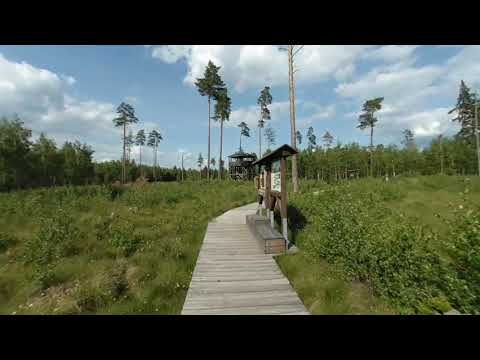The photograph captures a serene outdoor scene featuring a wooden plank path composed of equal-sized grayish planks that run straight before curving out of sight. Surrounding the path on both sides is lush green grass interspersed with small bushes and vegetation. Prominently in the foreground, there is a wooden signboard capped with a little roof, positioned behind a small, squat rectangular wooden bench. The signboard's content is unreadable due to the angle and distance. Above, the sky is a light blue adorned with multiple white, fluffy clouds, casting a warm, sunny glow that highlights the vibrant greenery. In the distance, a tree line includes a variety of trees with green leaves and notably taller palm trees with broad green tops, enhancing the picturesque nature of the setting. This peaceful scene, potentially set in a park or resort area, offers a tranquil walkway designed for pedestrian use.